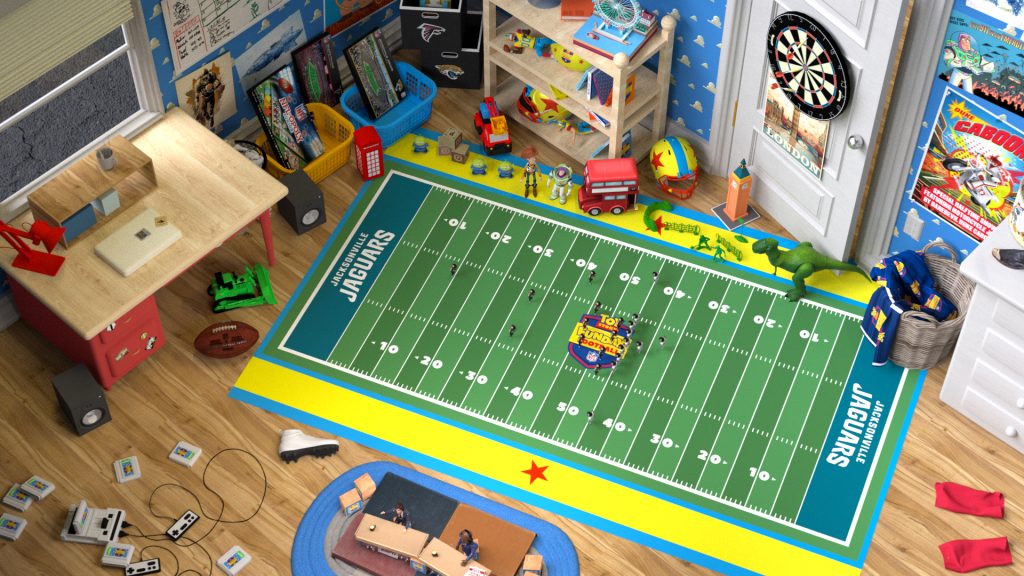This is an overhead photo of a vibrant child's playroom, taken from above, likely from a ceiling perspective or the second floor. At the center of the room is a mat designed like a football field, marked with ten-yard lines and white letters on a blue background that says "Jaguars," bordered by bright yellow sidelines with stars. The room features light-colored bamboo wood plank flooring. To the left, there is a small desk with a red desk lamp. Center right, at the top of the image, a partially open door reveals a dartboard with black and white design and several darts stuck in it. 

The room is filled with a variety of toys and games scattered around, including blocks in tubs, balls with stars, and remote-control gadgets with cartridge inserts. Notably, there's a dinosaur toy near the edge of the football mat and action figures like Woody and Buzz Lightyear from Toy Story. A hamper holding colorful blue and yellow pajamas can be spotted in the corner. Posters adorn the walls, adding to the playful and lively ambiance of the room.